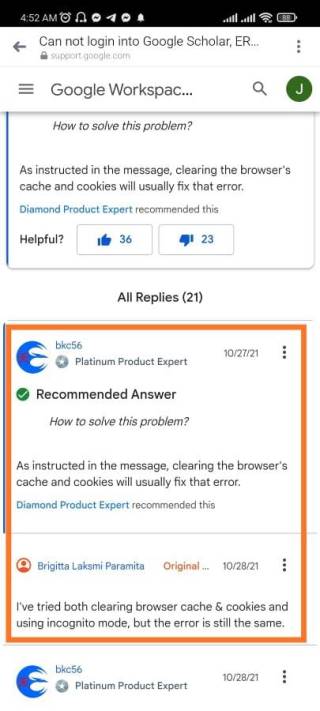This is a detailed caption for an image captured from an Android smartphone at 4:52 a.m. The image depicts various status icons at the top, including an alarm clock (indicating an active alarm), a headset symbol (signifying a plugged-in headset), two Facebook Messenger icons, a Telegram icon, a notification bell, two signal strength indicators (suggesting the use of dual SIM cards), and a Wi-Fi icon showing full connectivity. The battery icon indicates an 88% charge.

The central content of the screenshot is a discussion thread from Google Support, where users are addressing issues with Google Scholar. A highlighted message within the discussion suggests that clearing the browser's cache and cookies will usually resolve the specified error. This suggestion is endorsed by a user labeled as a "Diamond Product Expert." Directly below the expert's recommendation, there's an option for other users to indicate whether they found the advice helpful by clicking "yes" or "no."